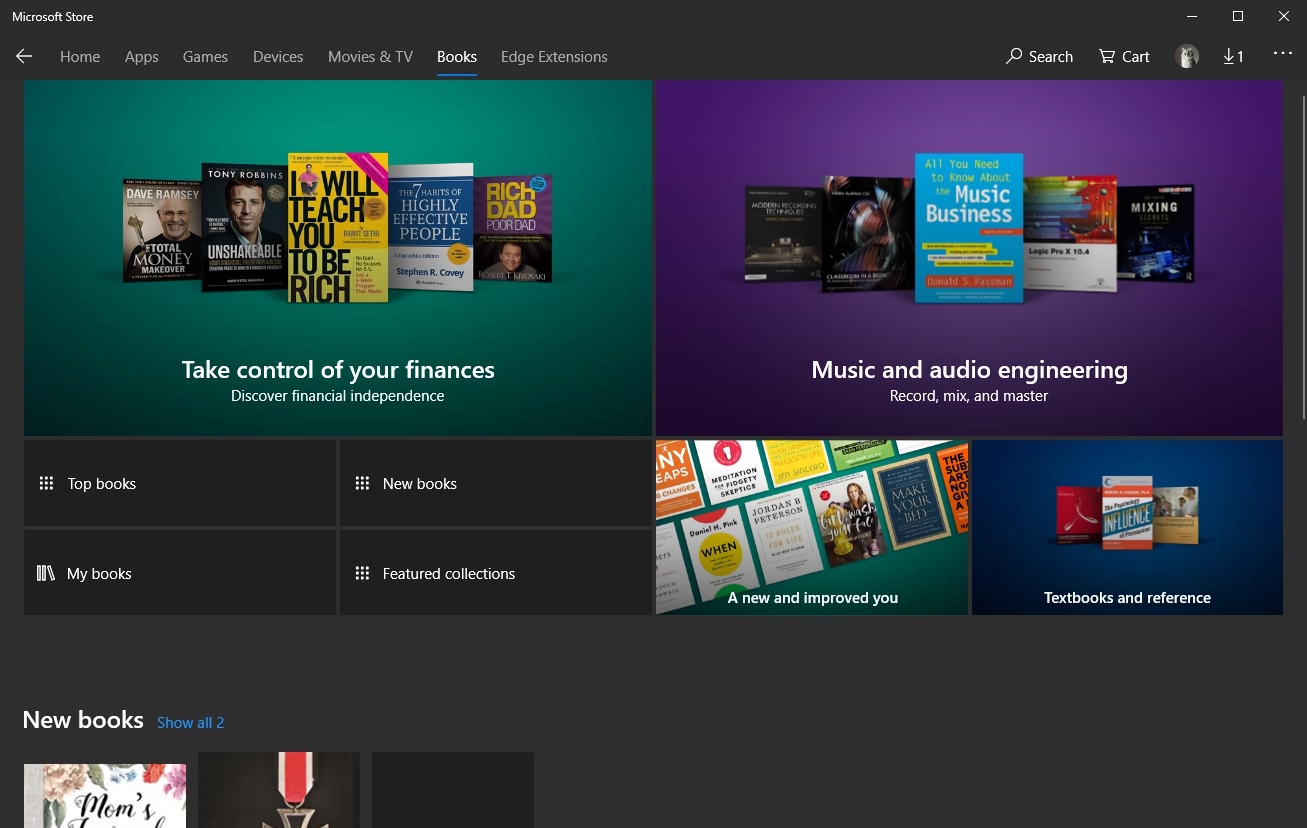The image showcases a section of the Microsoft Store interface. At the top, there is a black border with "Microsoft Store" at the top left, accompanied by an arrow pointing left. Next to it are the categories: "Home," "Apps," "Games," "Devices," "Movies & TV," "Books," and "Edge Extensions." On the top right, there is a search bar and an icon that says "Cart." Beside the cart icon, there is a profile picture that appears to be a cat, though it's small and unclear. There's also a download icon with the number one next to it.

Beneath this, on the left side, there’s a turquoise-colored section displaying a selection of books. Among them are "The Total Money Makeover" by Dave Ramsey, "Unshakeable" by Tony Robbins, "I Will Teach You to Be Rich," "The 7 Habits of Highly Effective People," and "Rich Dad Poor Dad." Below this collection of books is a text that reads, "Take control of your finances. Discover financial independence." Further below, there is a box with the labels "Top Books" and another that reads "New Books."